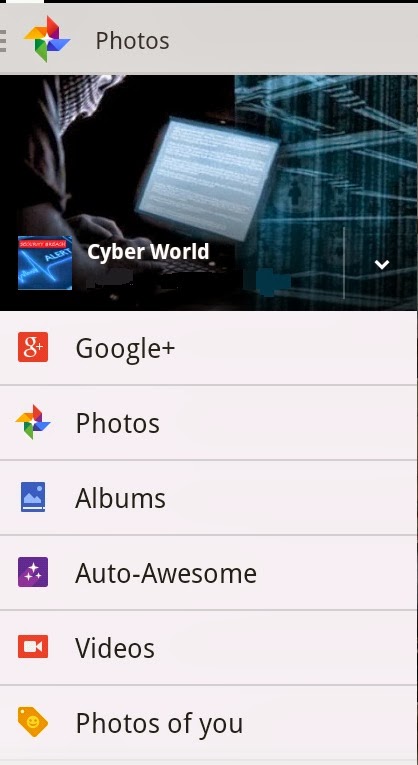**Detailed Caption:**

This image is a screenshot taken from a mobile device showcasing the Google Photos web application interface. The top half of the screenshot features a header bar with a gray or beige background. On the left side of the header, there is the iconic Google Photos pinwheel logo, composed of four leaves in the colors gold, green, blue, and red. Adjacent to the logo is the text "Photos" written in a clean, modern font.

Below the header, the main content of the screenshot includes an image on the left side, depicting a person seated and looking at a computer screen, which appears to be in dark mode with some white text displayed on it. Superimposed on this image is a thumbnail showing what resembles a medical alert graph or time series chart, characterized by red text and some white illegible text. The word "alert" is visible in blue on this thumbnail.

To the right of the overlayed image, the text "Cyberworld" is displayed, and on the extreme right side, there is a drop-down menu indicator. The background behind this section is predominantly black, with light blue outlines framing the interior of what looks like a multi-story building.

Beneath this section, six rows of apps or options are neatly listed. Each row includes an icon to its left:
1. **Google+:** Represented by the red square "G+" logo.
2. **Photos:** Denoted by the familiar Google Photos pinwheel logo.
3. **Albums:** Illustrated by a blue icon portraying an image with a line beneath it, featuring mountains and a sun in lighter blue shades.
4. **Auto Awesome:** Signified by a purple background with three white four-point stars.
5. **Videos:** Marked by a white video camera icon atop an orange rectangular background.
6. **Photos of You:** Identified by a yellow tag with a smiley face inside it.

This detailed interface provides users with various options to access different features within the Google Photos ecosystem.